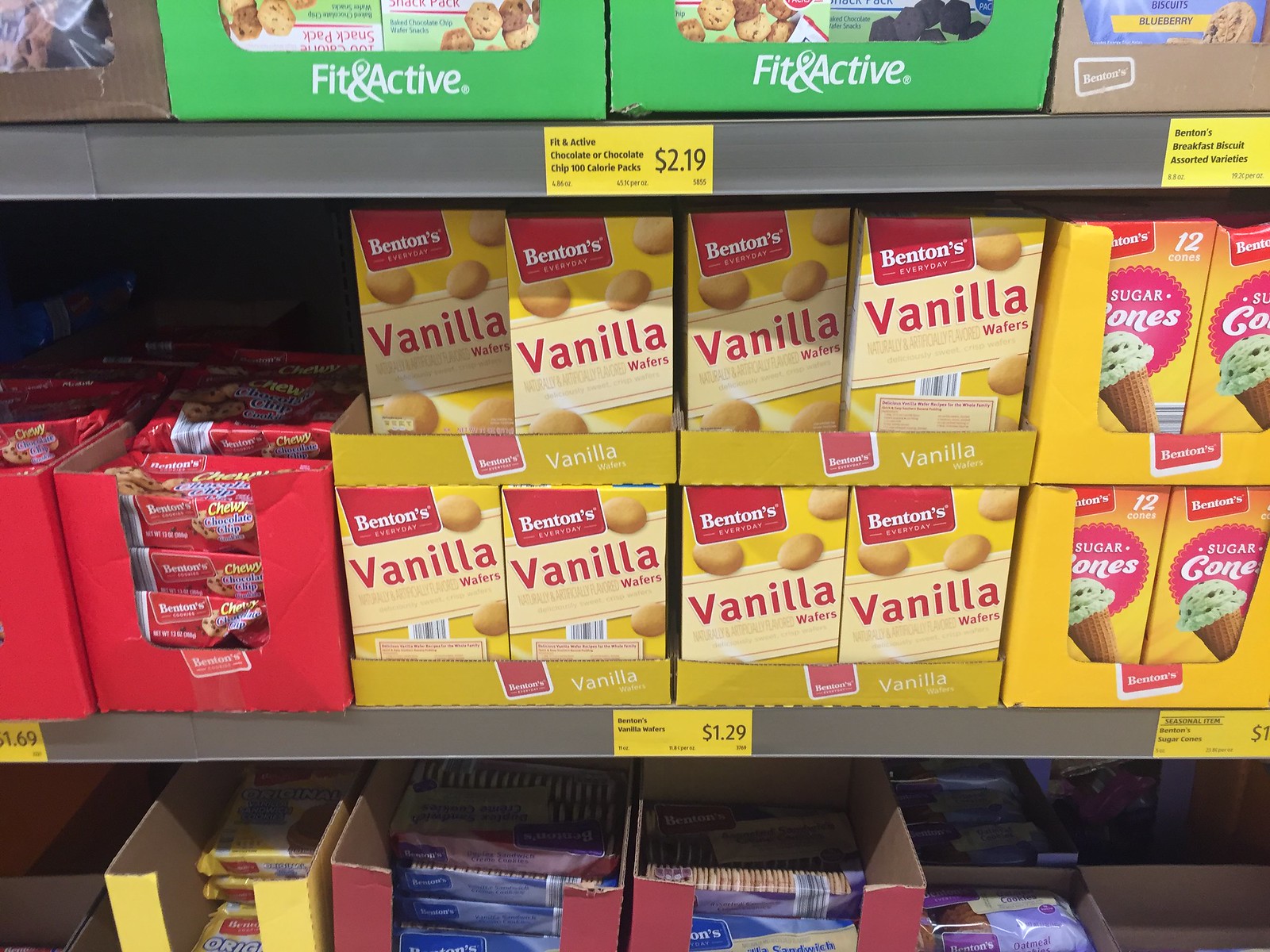The image depicts a close-up of grocery store shelves, likely taken inside an Aldi. The shelves are gray and display a variety of boxed foods. On the top shelf, there are green boxes labeled "Fit and Active" priced at $2.19, alongside brown boxes of Benton's cookies. The middle shelf prominently features yellow boxes of Benton's Vanilla Wafers priced at $1.29, with some sugar cones in red and yellow packaging nearby. The bottom shelf shows a mix of cookies in purple and yellow packaging. Overall, the shelves are neatly organized with clear yellow price labels and black lettering, showcasing a range of cookie and snack options.